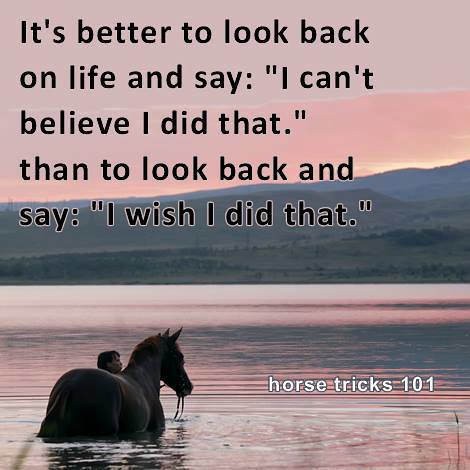This vividly detailed poster captures a serene scene at dusk, portraying a picturesque landscape awash in varying shades of pink, purple, blue, and hints of yellow-orange. A man and a horse stand partially submerged in a calm lake or river, with the horse chest-deep in water. The man's head is visible behind the horse, both appearing to gaze thoughtfully into the distance. In the background, the distant horizon features rolling hills that blend seamlessly with the colorful sky, reflecting similarly hued tones onto the water's surface. Prominently, a motivational quote near the top of the poster reads, "It's better to look back on life and say I can't believe I did that, than to look back and say I wish I did that," in bold black print. The lower right corner of the image is marked with the white text, "Horse Tricks 101." The harmonious blend of colors and elements creates a tranquil yet inspiring visual that evokes both contemplation and a sense of adventure.